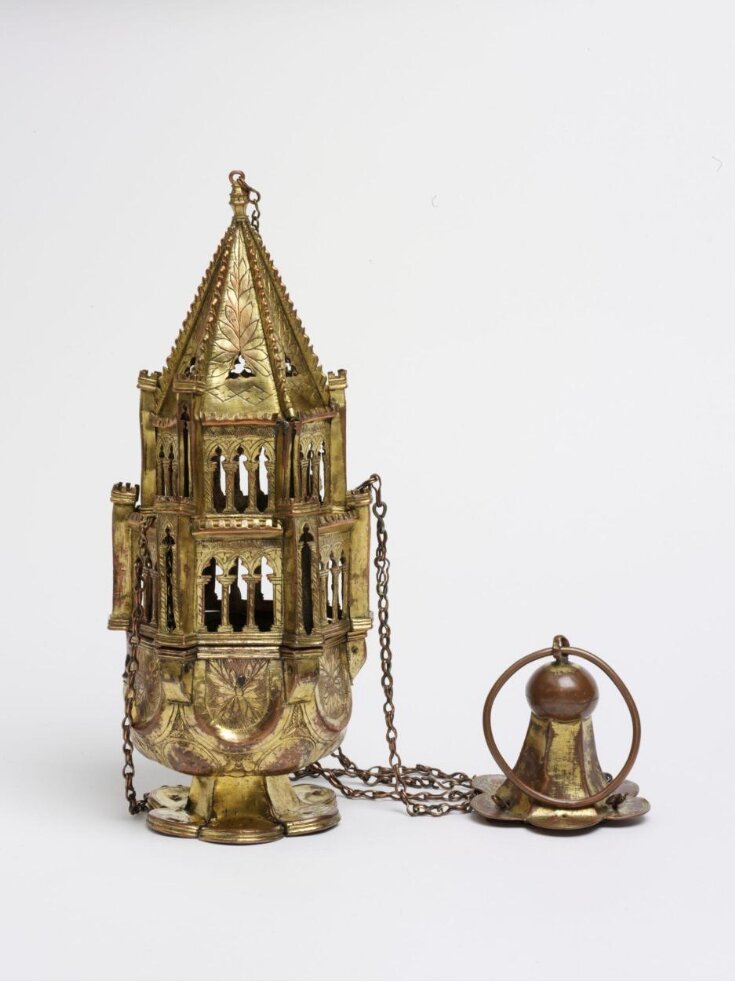This is a color photograph of an ornate, vintage gold artifact, likely a thurible used in Christian worship to spread incense. The artifact, intricately designed with floral patterns and gothic detailing, is divided into two main parts connected by a series of chains. The primary section resembles a miniature gothic cathedral or tower with a steeply pitched roof and two rows of windows, all rendered in a gold-brass hue. The secondary part, attached to the chains, features a fluted metal cone-shaped floral cap with a circular ring on top, suggesting it can be hung or used manually. This exquisite piece, sitting against a white background, showcases remarkable craftsmanship through its carved detailing and interconnected structures.